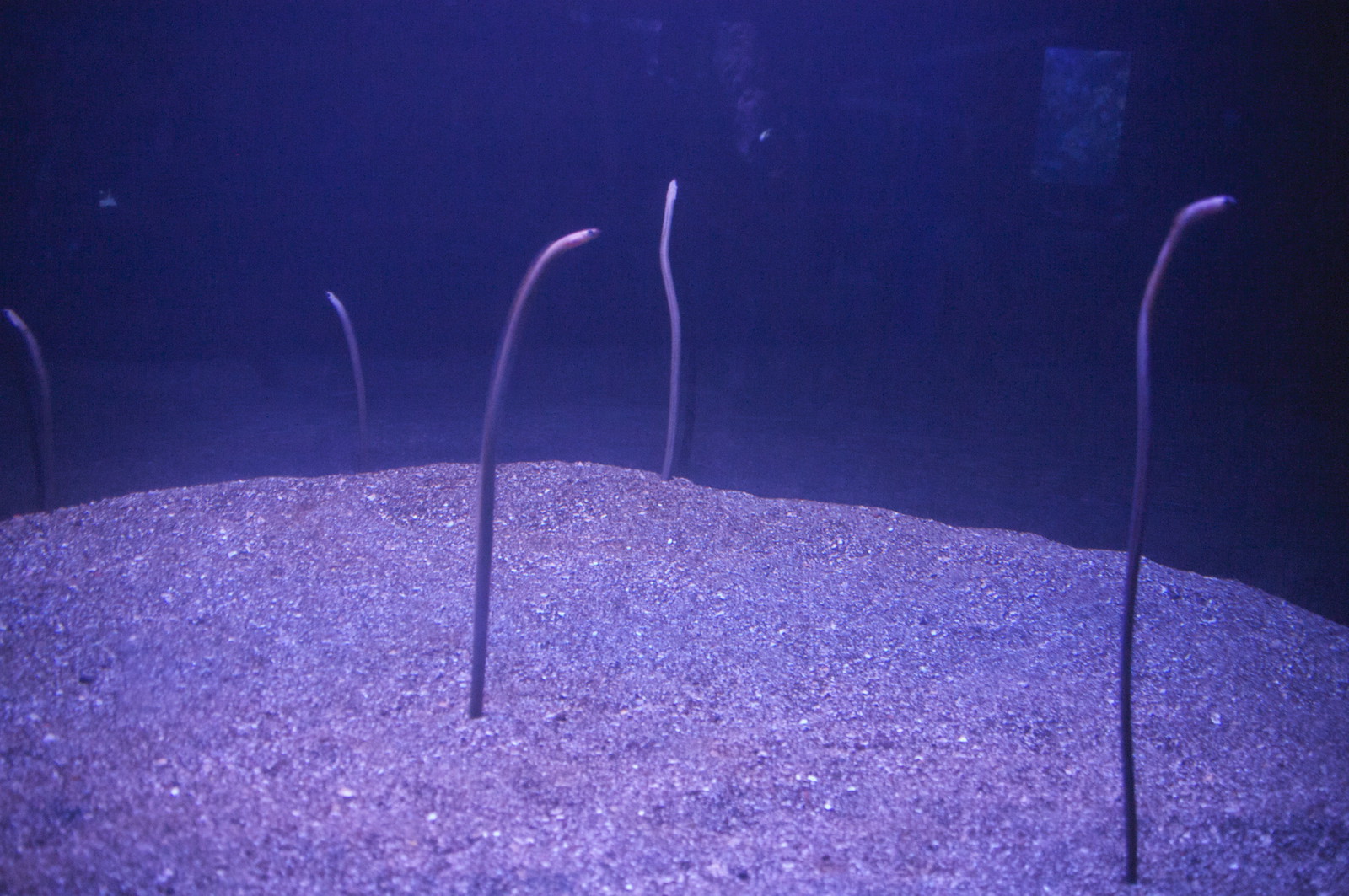The image depicts an underwater scene that might be either a photograph from inside an aquarium or a computer-generated visual. The overall hue of the image is a blend of blue and purple tones, contributing to a serene aquatic ambiance. The upper section of the image is dominated by dark, deep bluish-purple water, while the bottom portion showcases a sandy area that transitions smoothly like a gentle hill. This sand is tinged with pinkish and blue hues.

In this sandy expanse, five slender, eel or worm-like creatures are protruding vertically, as though standing on their tails embedded in the sand. These creatures, copper-colored and thin, appear to have eyes at their tips and are spaced across the image; three are situated further in the background, while one is centrally located and another positioned near the bottom right. The reflective quality of the scene suggests a glass barrier, hinting at an aquarium setting, and there are reflections visible near the top of the image, contributing additional depth and detail.